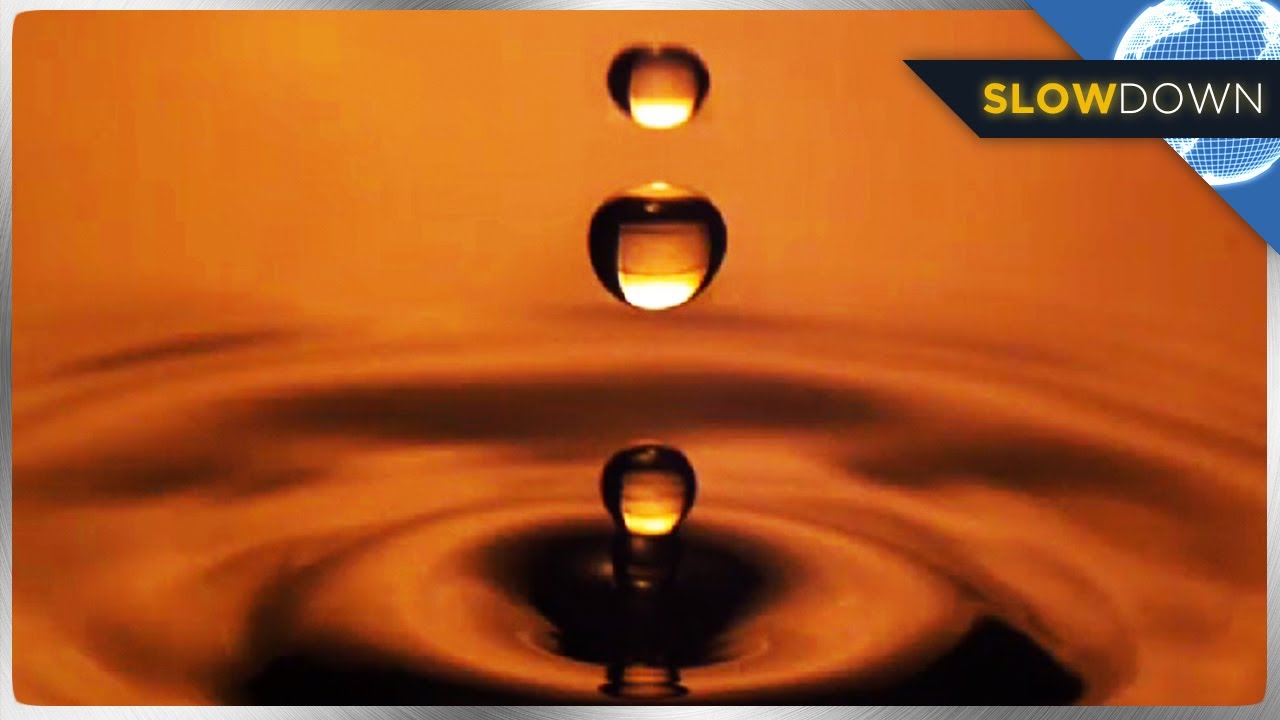This photograph captures the mesmerizing mid-motion of three high-speed water droplets aligned vertically against a warm orange-yellow background. The central droplet is the largest, flanked by two slightly smaller droplets at the top and bottom. The scene includes a visible ripple effect where the droplets interact with a small puddle below, adding a dynamic sense of motion. Enhancing the composition is a metallic silver border framing the image. In the upper right corner, a globe with a grid-like design and a black ribbon banner displays the words "SLOW" in yellow and "DOWN" in white, suggesting perhaps a stock or company image with a message encouraging deceleration. The droplets, glistening in gold hues at the top and transitioning to lighter tones towards the bottom, create a striking visual akin to droplets falling into a creamy liquid, reminiscent of coffee or pudding.